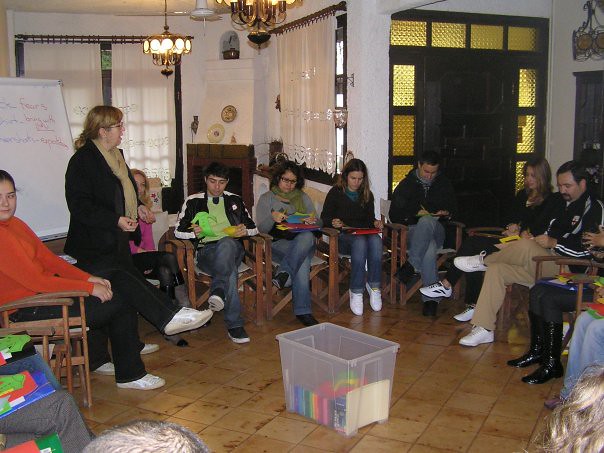This square photo captures a group of around twelve people gathered in a room, seated in a roughly circular formation on small wooden chairs. They seem to be engaged in a study group, attentively listening to a woman standing on the left side of the image. The woman is wearing black pants and a black blazer over a gold shirt, with her hands gesturing as she speaks. The room features a brown tile floor with darker brown accents, and the upper right corner shows a black wooden door framed by small gold-tinted window cutouts. Nearby, a white dry-erase board with illegible writing is positioned. The left side of the room is backed by white-curtained windows and illuminated by a chandelier casting a white light. In the center of the room, a clear bin filled with colorful books stands out. Most attendees are dressed casually in denim jeans, each with a writing pad in their laps, contributing to a focused and attentive atmosphere.